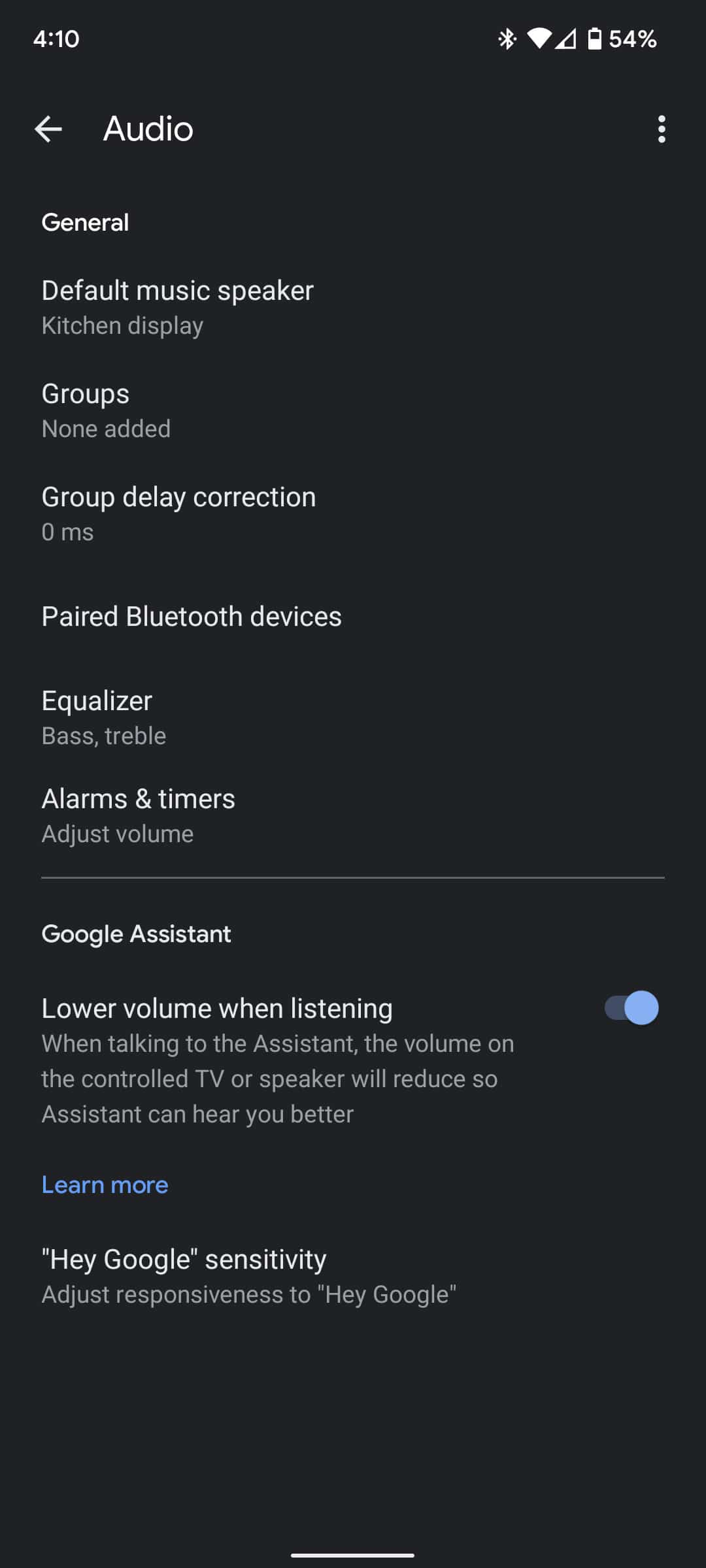This is a detailed screenshot taken from a cell phone at 4:10, as indicated by the timestamp in the top left corner. The battery level in the top right corner shows 54%. The entire background is black with white text. 

At the very top, in the upper left corner, the word "Audio" marks the section of the control panel within a particular cell phone app. Just below it, another section titled "General" includes various settings. The default music speaker is set to "Kitchen Display," and it indicates that no groups have been added ("Groups: None Added"). The "Group Delay Correction" is set to 0 ms. The section for "Paired Bluetooth Devices" shows no devices listed under it. The "Equalizer" settings display options for adjusting bass and treble. Following this are settings related to "Tones and Timers," with the prompt "Adjust Volume" situated below it.

A light gray line divides these sections from the "Google Assistant" settings below. The "Google Assistant" section includes a description and a toggle button to the right. The toggle for "Lower volume when listening" is switched to "On." The text under this setting explains that when talking to the Assistant, the volume on the controlling TV or speaker will reduce to better hear the user's commands. This section also includes a "Learn more" link for additional information.

At the very bottom of the screenshot, there is a setting titled "Hey Google Sensitivity," which allows adjustments to the responsiveness of the "Hey Google" command.